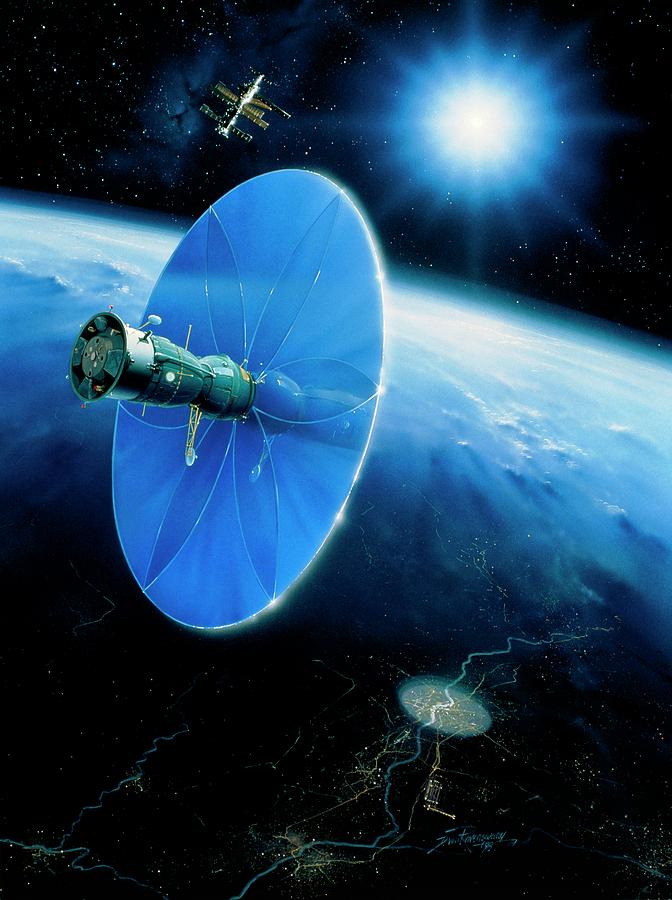In this striking digital artwork, the viewer finds themselves orbiting the Earth amidst the dark, boundless expanse of space. At the bottom of the image, the Earth is depicted in a striking black and blue, punctuated with small light dots that represent illuminated areas. Notably, there is a satellite with a prominent mirror on its front, angled towards the Sun, and this reflection appears to illuminate a portion of the Earth below, revealing an oval-shaped river in the night landscape.

This particular satellite is mostly green with a round front part, rocket nozzles at the rear, and a strip of metal near the top. A small green protrusion sticks out just before the rocket nozzles. In addition to this, another satellite at the lower right corner appears to be emitting what look like laser beams or bolts of electricity.

Above the Earth, the viewer sees the radiant Sun to the top left, shining with a mix of white and blue light, radiating visible rays against the pitch-black void of space which is dotted with countless star-like white specks. In the backdrop, the vast, star-filled universe serves as a serene contrast to the dynamic elements of the scene.

Additionally, a space station is observed slightly above the curvature of the Earth, featuring a central core with several protruding modules. Despite the Sun seeming distant, its light—or possibly the reflection from the satellite mirror—illuminates parts of the station, making its structure visible against the inky blackness of space. The composition of the scene suggests a seamless transition between the illuminated and shadowed regions of Earth, highlighting the mesmerizing juxtaposition of night and day on the planet below.